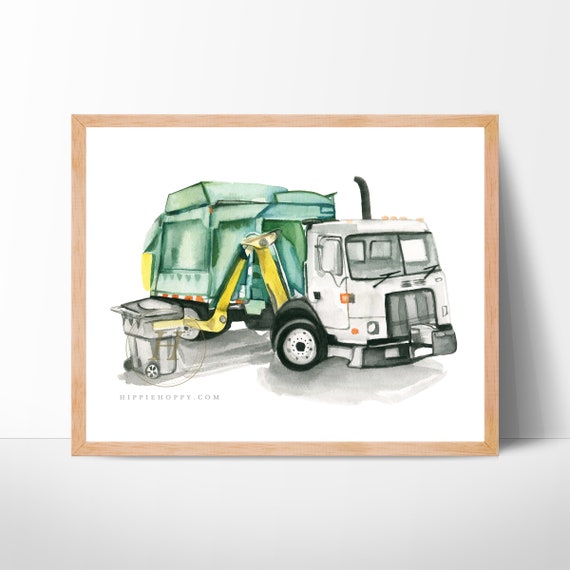The image displays a detailed watercolor painting of a garbage truck, positioned within a wooden frame that has light brown, thin edges. The composition of the photo inclines from a white upper left-hand corner background to a light gray shade in the lower right-hand corner, likely influenced by the light source. The depicted garbage truck faces right and offers a view of the front-right section, showcasing its white cab and green dump area. Prominently, two yellow mechanical arms extend from the side, engaging with a gray, wheeled trash can labeled with "hippie.com" underneath. The scene is set against a white background, and the entire framed artwork leans against a white wall, placed on a cream-colored floor.